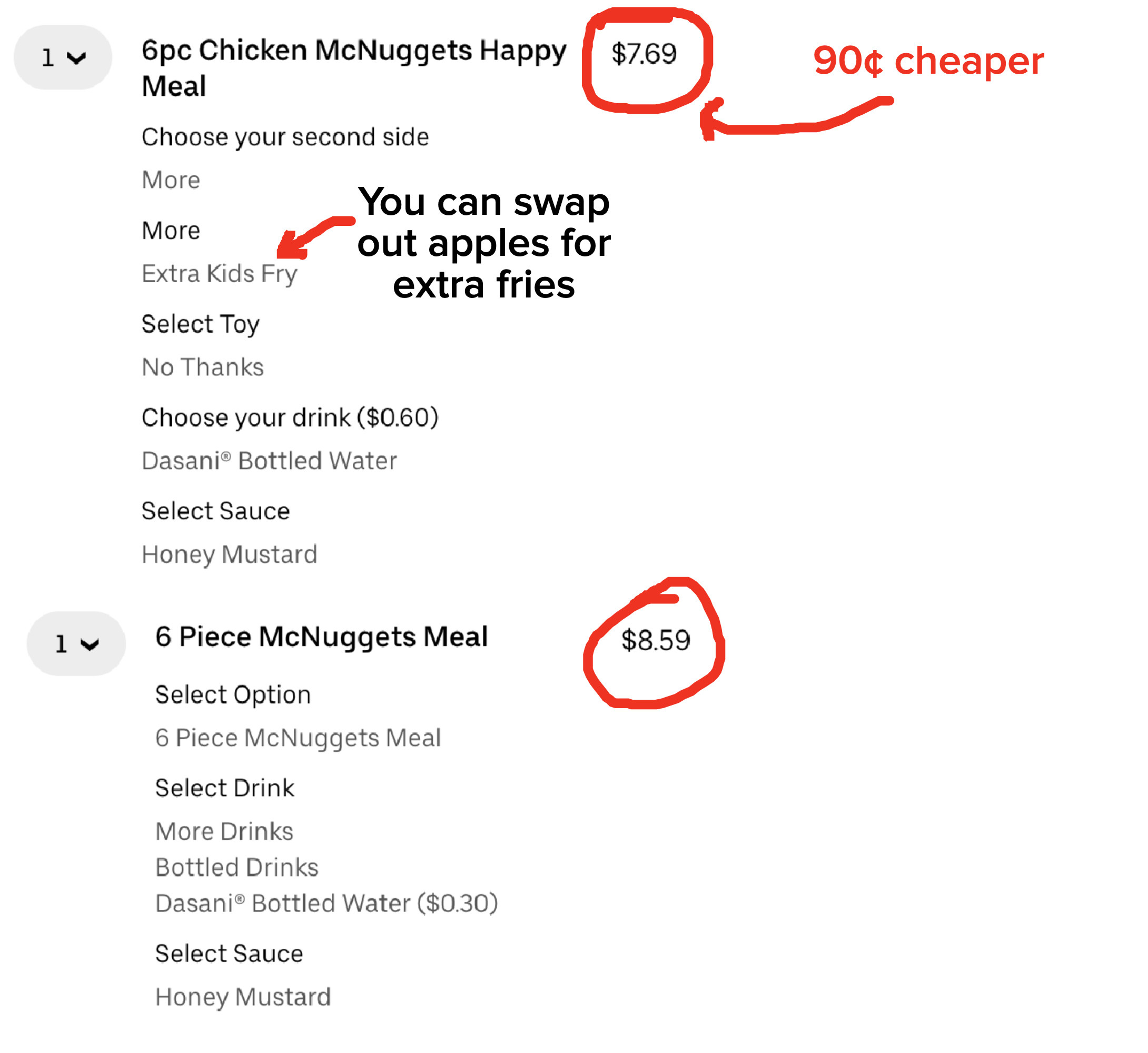The image displays a digital menu screen detailing the order process for a McDonald's 6-piece Chicken McNuggets Happy Meal. At the top, there's a dropdown menu labeled "1" indicating the quantity. Below, it lists the meal at $7.69, which is highlighted with a red square. To the right, red text points out that the meal is "90 cents cheaper" with an arrow pointing to the price. Further options appear beneath, including "Choose your second side" with an option to swap apples for extra fries, labeled "Extra kid fries". The "Select toy" section shows "No thanks" as the selected option. For drinks, "60 cents" is displayed next to "Dasani bottled water". The sauce selection is highlighted with "Honey Mustard" chosen. Further down in the image, another section shows the 6-piece McNuggets meal priced at $8.59, highlighted with a red circle. It includes similar customization options: choosing a drink from a dropdown menu, indicating more drink options including bottled drinks, specifically "Dasani bottled water" for an additional 30 cents, and selecting "Honey Mustard" sauce again.